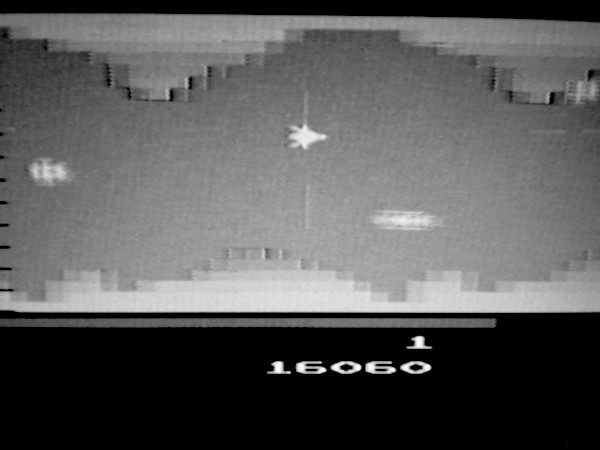A grayscale screenshot from a computer game's action sequence. The image features a jet maneuvering through a hazardous course filled with flying objects that the player must either dodge or shoot down. The game interface is stylized with pixelated, stepped pyramidal shapes flanking the sides of the screen, framing the jet's flight path. At the bottom of the screen, bold black text is displayed against a black background, showing the player’s current score of 16060 in contrasting white.